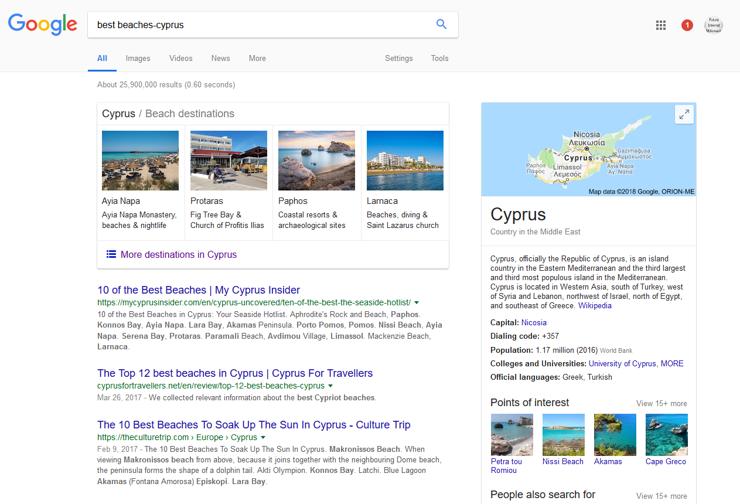A screenshot of Google search results for the query "best beaches, Cyprus". The left side of the screen displays the Google logo in blue, red, yellow, and green, followed by the search bar with the entered query. Beneath the search bar, there are tabs labeled 'All', 'Images', 'Videos', 'News', and 'More', with the 'All' tab selected and highlighted in blue, while the others remain gray. A blue line underscores the 'All' tab. The search returned approximately 25,900,000 results in 0.60 seconds.

The top section showcases beach destinations in Cyprus, accompanied by four photos labeled "Ayia Napa", "Protaras", "Paphos", and "Larnaca". Below the images, a link directs users to more destinations in Cyprus.

Further down, the search results list begins with the following entries:
1. "10 of the Best Beaches" by My Cyprus Insider.
2. "10 of the Best Beaches in Cyprus".
3. "Top 12 Beaches in Cyprus" by Cyprus for Travelers.
4. "10 Best Beaches to Soak Up the Sun in Cyprus" by Culture Trip (theculturetrip.com).

All results appear to be from 2017.

On the right side of the screen, an overview panel features a map of Cyprus with a brief description, identifying it as a country in the Middle East.